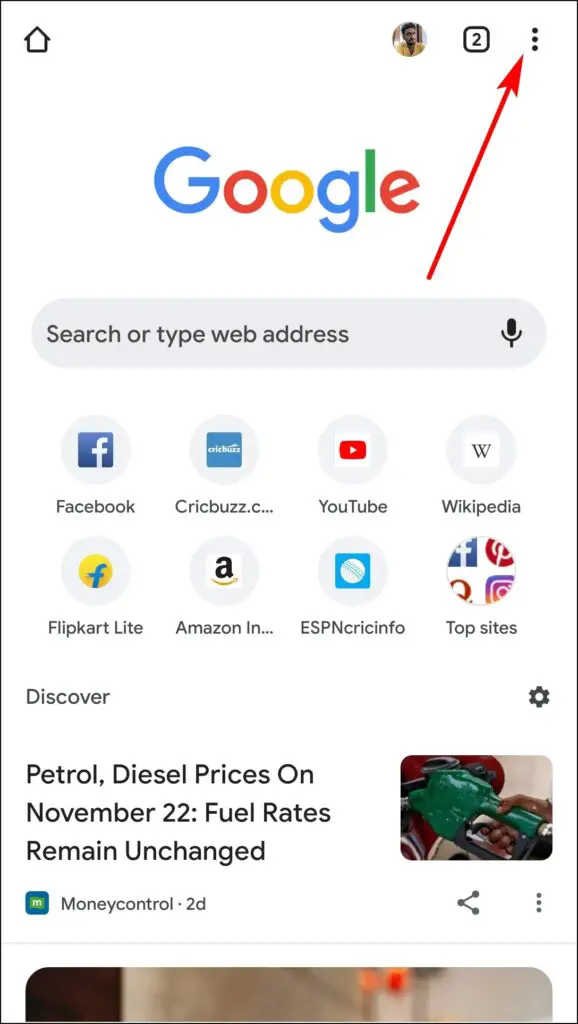A person is using Google search on their smartphone. The screen displays a large red arrow pointing to the three vertical bar menu icon in the top-right corner, for reasons unknown. In the top left, there's a home button, while a profile picture of a man's face is visible next to a square icon with a number 2 inside, indicating two open tabs.

Central to the screen is the prominent Google logo, positioned above a search field in a capsule design. The search field prompts "Type web address," and features a microphone icon to its right.

Beneath the search field, there are eight app icons arranged in two rows of four: Facebook, Quick Buzz, YouTube, Wikipedia, Flipkart Lite, Amazon, ESPN, and Top Sites, each with their respective logos displayed above the text labels.

Further down, the interface shows a "Discover" section with a gear icon on the right side, typically used for settings. An article is partially visible below this with a photo on the right, depicting a close-up of a hand holding a green-handled gas pump nozzle. Accompanying the image, the text reads: "Petrol/Diesel prices on November 22nd; fuel rates remain unchanged," attributed to Money Control from two days ago. Below this article snippet are a share icon and an additional three-dot menu.

At the very bottom of the screen, there is the top portion of another full-width image, which appears to be cut off, requiring scrolling to view the rest of it. Its content is unclear from the visible portion.